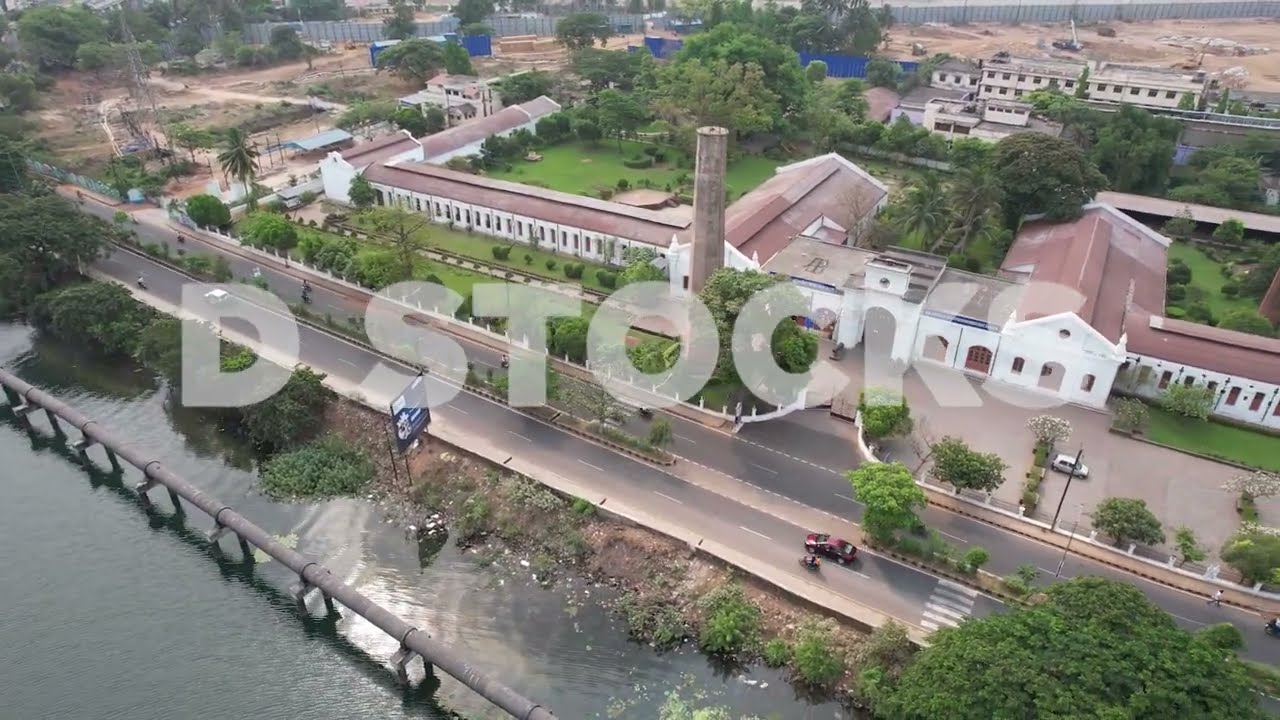The photograph captures an outdoor scene in a city during daylight. In the lower left-hand corner, a river runs diagonally from the center bottom to the upper center left, crossed by an elevated grey pipeline. Beyond the river, a sandy or dirt embankment is dotted with green bushes and trees. On top of this embankment, a two-lane road extends, with a central median separating the directions. To the left side of the image, a dirt area is scattered with green foliage.

Dominating the upper right-hand side is a long, single-story white building featuring two main wings that appear to contain large courtyards filled with green trees. This building, resembling an old Spanish ranch house or perhaps a church, seems suited for institutional use, possibly with spaces such as auditoriums or meeting rooms. Adjacent to this structure, more buildings are visible in the background along the horizon line, with some larger structures toward the left.

A watermark with the text "D. Stocks" or "DSTOC" spans across the center of the image in transparent white block print.